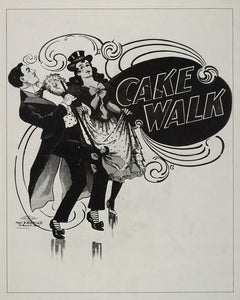The image is a vintage-style black and white poster in a portrait layout, featuring an off-white, cream background bordered by a thin black line. Within this border is a drawing of a man and a woman dressed in formal, somewhat theatrical attire. The man is in a tuxedo with short, neatly combed hair, a neatly trimmed mustache, and striped socks, holding a cane. The woman, wearing a top hat, has long black hair and is dressed in a long, white polka dot skirt with a black corset adorned with a ribbon design. She holds up her skirt, revealing her black socks and heeled shoes. Both are depicted in animated dance poses with their knees raised, seeming to prance in a lively manner.

To the right of the couple is a prominent black circle containing the text "CAKE WALK" in bold, white, all-capital letters spread over two lines. Surrounding the couple and circling around the black circle are intricate, swirling design elements that add a sense of movement and flair to the image. Despite being monochromatic, the shading effectively defines the details and adds depth to the poster. There is no other text or color featured in the image.